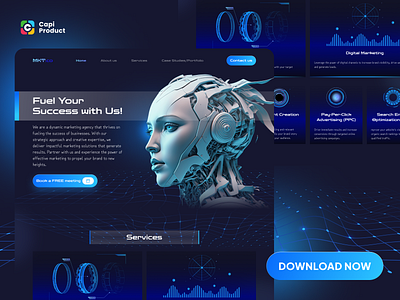The image depicts an advertisement on a computer screen with a very dark blue background, accented by various shades of blue lettering and some yellow text. Dominating the center is an intricate, stylized drawing of a woman with metal components and wires composing her head. Her face, smooth with blue eyes, contrasts with the metallic shreds that form her hair and the exposed mechanical parts of her brain. A large circular device replaces her ear, resembling a speaker. Above her head, a gray and white banner reads, "Fuel your success with us." To the right of her image, there are interactive elements, including charts and rings, indicative of additional information or options related to the advertisement. The upper left corner features white text stating "CAPL product" beside a colorful square logo. The bottom right corner contains a call-to-action button that says "Download Now." Various sections, like one labeled "services," also appear on the page, suggesting clickable content.